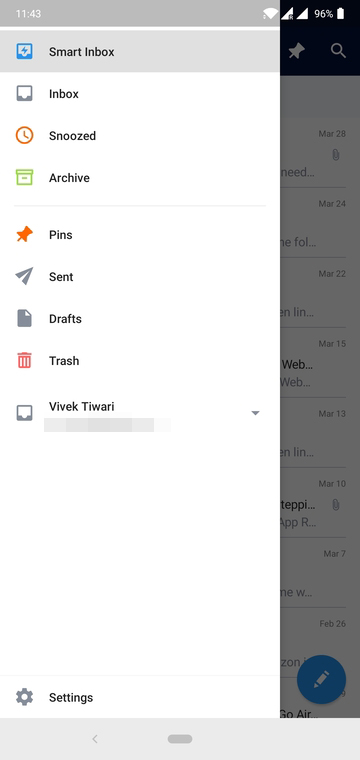The screenshot depicts an interface from what appears to be an iPhone. In the background, there's a faint glimpse of a document or another app partially visible on the right edge, extending vertically from top to bottom. The main focus of the screenshot is a large white menu pop-up originating from the left side and covering about four-fifths of the screen’s width.

This menu is sequentially organized with various selectable items each accompanied by a distinct icon. The list starts with "Smart Inbox" highlighted in blue, indicating that it is currently selected. Below it are:

1. "Inbox" in standard text.
2. "Snoozed" marked with an orange clock icon.
3. "Archive" paired with a green file container icon.
4. "Pins" featuring a red pin icon.
5. "Sent" indicated by a gray paper airplane icon.
6. "Drafts" with a gray dog-eared page icon.
7. "Trash" signified by a red trash can icon.

At the bottom of the menu, the user's name "Vivek Tiwari" is displayed, likely denoting the account owner. The overall interface appears to be a well-organized email or message management application.